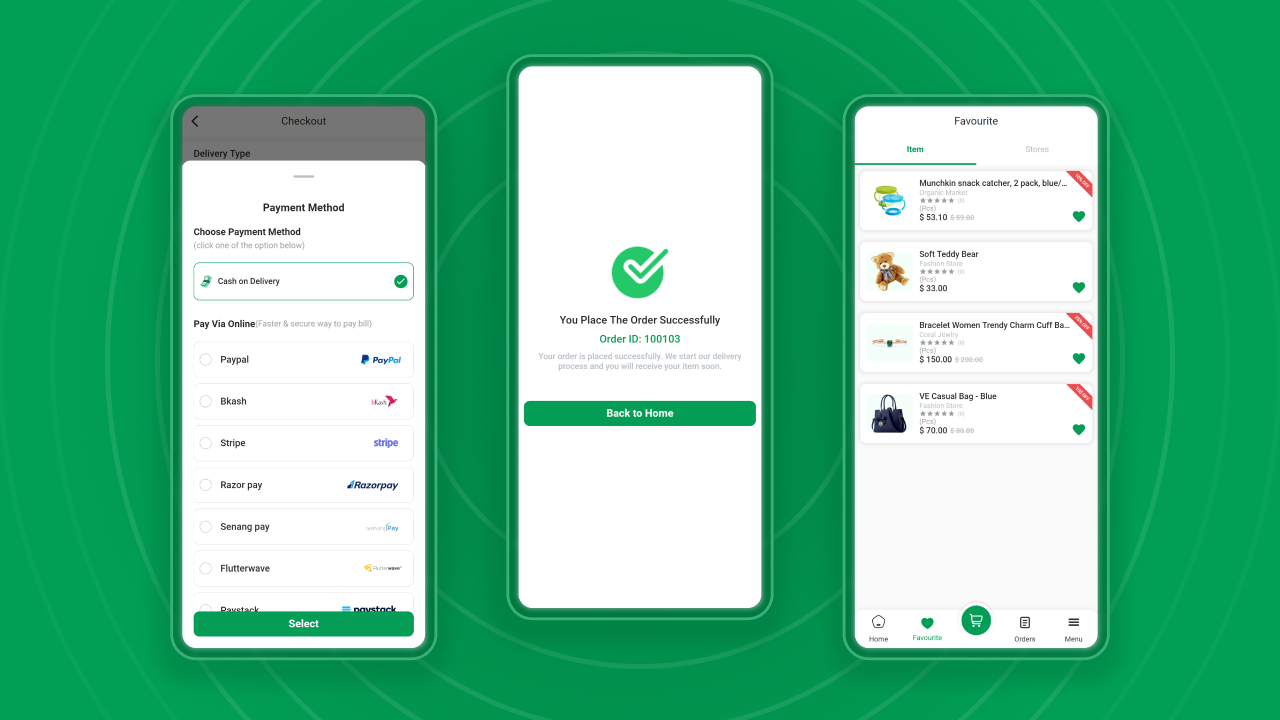The image consists of three sequential screenshots related to an online purchase transaction. 

1. **Left Screenshot**: The first screenshot illustrates the payment method selection screen of an online shopping platform. The options for payment methods are clearly listed as "Cash on Delivery" and several online payment options including PayPal, Bcash, Stripe, Razorpay, ZenoPay (a lesser-known service), Flutterwave, and Paystock. The user has opted for "Cash on Delivery."

2. **Middle Screenshot**: The second screenshot features a confirmation screen with a green check mark, indicating the successful placement of the order. It includes an order ID of "100103" and a message stating, "Your order is placed successfully. They'll send you delivery information." A button labeled "Back to Home" is also visible, allowing the user to return to the main interface.

3. **Right Screenshot**: The third screenshot displays the "Favorite" section, highlighting selected items. Visible items include two decorative bowls, a plush teddy bear, a women's bracelet, and a stylish purse.

This detailed visual sequence provides a comprehensive overview of the user's transaction journey, from selecting a payment method to order confirmation, and finally reviewing favorite items.